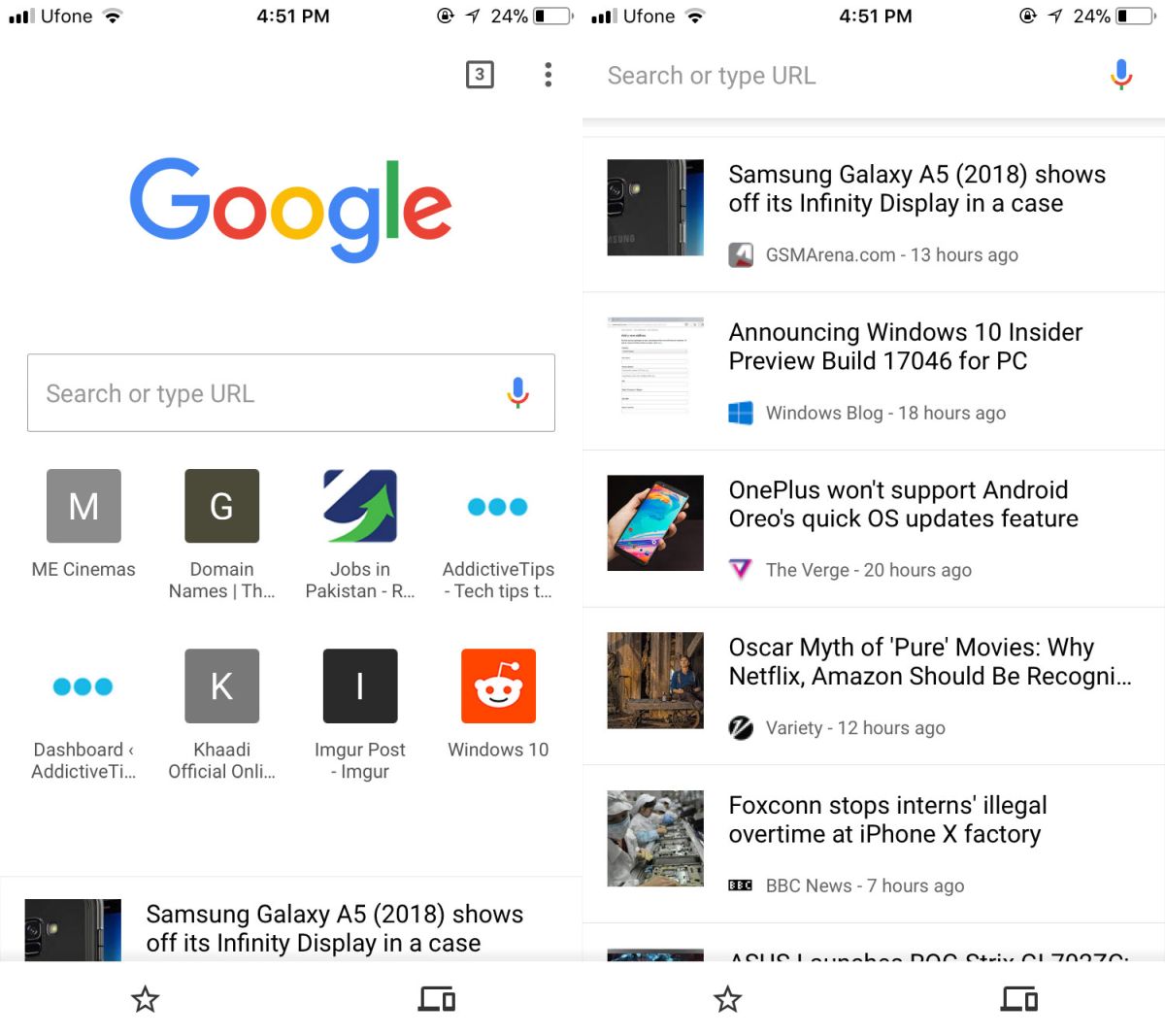At the top-left corner of the image is the iconic Google logo, featuring the letter 'G' in blue, the first 'O' in red, the second 'O' in yellow, the second 'G' in blue, an 'L' in green, and an 'E' in red. Directly below the logo is a search bar for typing in queries or URLs.

Below the search bar are eight symbols representing previously visited websites, arranged in two rows of four:

1. **MECinemas** - showing an 'M' logo.
2. **Donate Names** - featuring a black background and a vertical line.
3. **Ledger's TH** - simply labeled with text.
4. **Jobs in Pakistan** - depicted with a green arrow and a blue background intersected by a white line.
5. **Addictive Tips/Dash Tech Tips** - on a white background with three turquoise colored dots; the text trails off with an ellipsis.
6. **Coddy Official Online** - a white letter 'K' on a gray background.
7. **Imgur Post-Imgur** - with an 'I' on a black background.
8. **Reddit (Windows 10)** - identifiable by its orange background.

Underneath these symbols, a snippet details an article about the "Samsung Galaxy A5 2018" showcasing its display in a case. To the right, there are links to additional websites, revealing more browsing history:

- Samsung Galaxy A5: Announcing its features.
- Windows 10 Insider Preview Build: A link from the Windows Blog.
- OnePlus: Mentioning the lack of support for Android or RailsQuick OS update features, from The Verge.
- **Oscar Myth of Pure Movies**: An article from Variety discussing why Netflix and Amazon should be recognized.
- **Foxconn stops interns' illegal overtime at iPhone X factory**: News from BBC News.

The overall image is an organized snapshot of browsing history, encapsulated within the familiar Google interface.